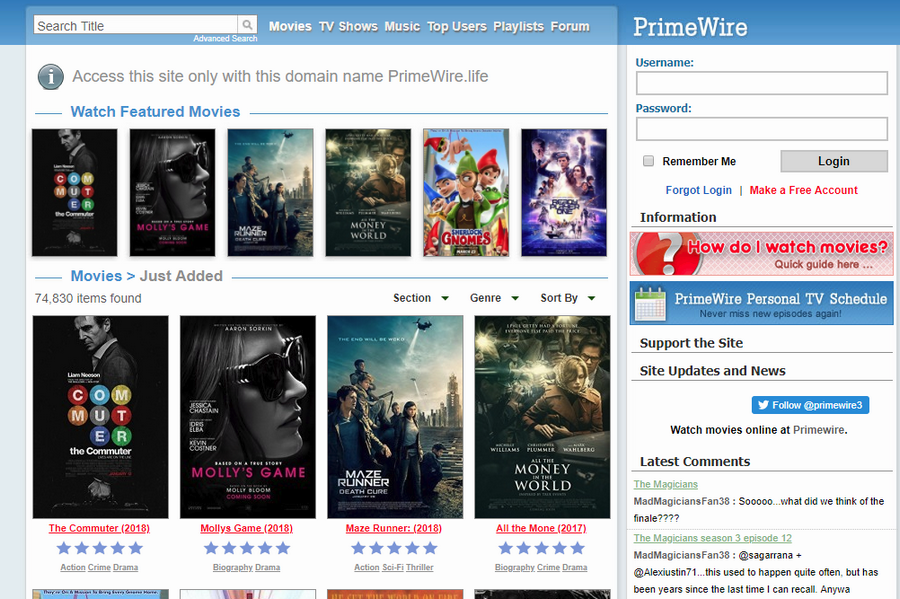This image depicts the homepage of a streaming website called PrimeWire. Dominating the layout are numerous movie posters, showcasing a diverse selection of films. On the right-hand side, there is an account login section, followed by an informational segment highlighted in bright red. This section features a quick guide to help new users navigate the site more efficiently.

Further down, information on supporting the site, recent updates, and user comments are prominently displayed. On the left-hand side, a search bar allows users to look up specific titles. Below this, navigational tabs provide quick access to categories such as Movies, TV Shows, Music, Top Users, and Playlists, alongside a forum. There is also an important note advising users to access the site exclusively through the domain name primewire.life.

The site promotes its featured movies, including titles like "Molly's Game," "Maze Runner," "All the Money in the World," and an animated film about gnomes. A prominent purple poster is also among the featured movies. Additionally, larger thumbnails of these films appear under the "Movie Section," which boasts an impressive catalog of 74,830 items. This suggests that PrimeWire offers an extensive library of content, likely for streaming rather than downloading.